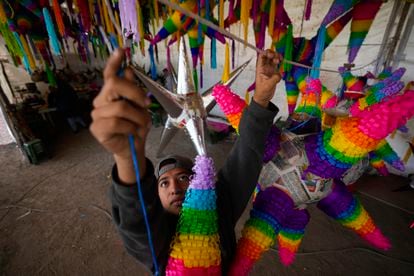The image shows a young man, possibly Mexican, viewed from above as he stands in a room filled with vibrant piñatas. He is wearing a dark gray sweatshirt and a backwards gray baseball cap. With both hands raised, he appears to be either hanging or arranging the piñatas on strings that drape from wall to wall or the ceiling. The piñatas are colorful, resembling multi-pointed stars with a central round body and cone-shaped foil arms, decorated in rainbow hues of pink, orange, yellow, green, blue, and purple. Some piñatas are adorned with dangling streamers in matching colors. Among the multitude, one piñata visibly waits to be decorated, only featuring silver spiky points. Behind and above the man, additional colorful strips of blue, red, yellow, orange, and white hang, adding to the festive atmosphere.